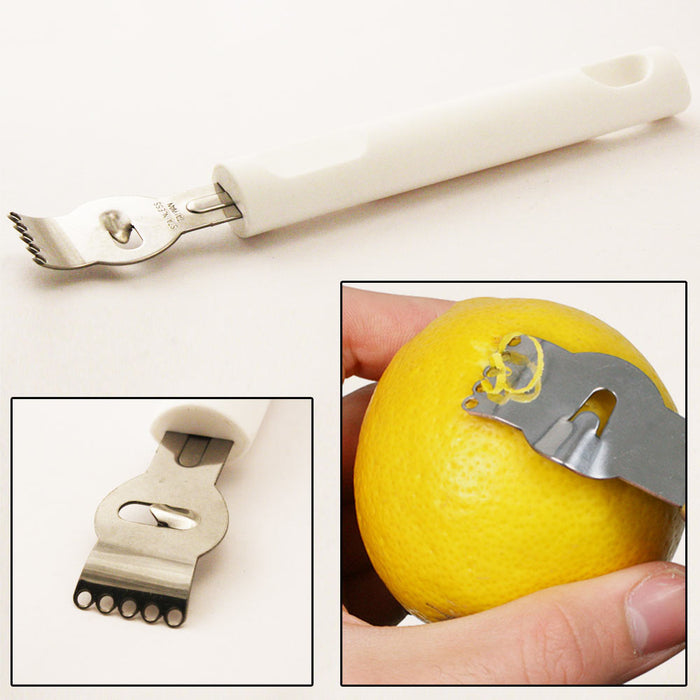The image is composed of three sections on a cream-colored background, presenting a detailed display of a lemon peeler. The top part showcases the entire handheld device, featuring a long, thin white handle with a steel head that resembles a combination of a can opener and a fork, including prongs and a bottle opener-like circular opening in the middle. The bottom left section contains a close-up of the steel head, illustrating the intricate design of the prongs and circular elements. The bottom right section depicts the lemon peeler in action: a left hand holding a lemon while the peeler scrapes the rind, producing spirally and circular lemon zest. This triptych image effectively highlights the product's design and functionality.